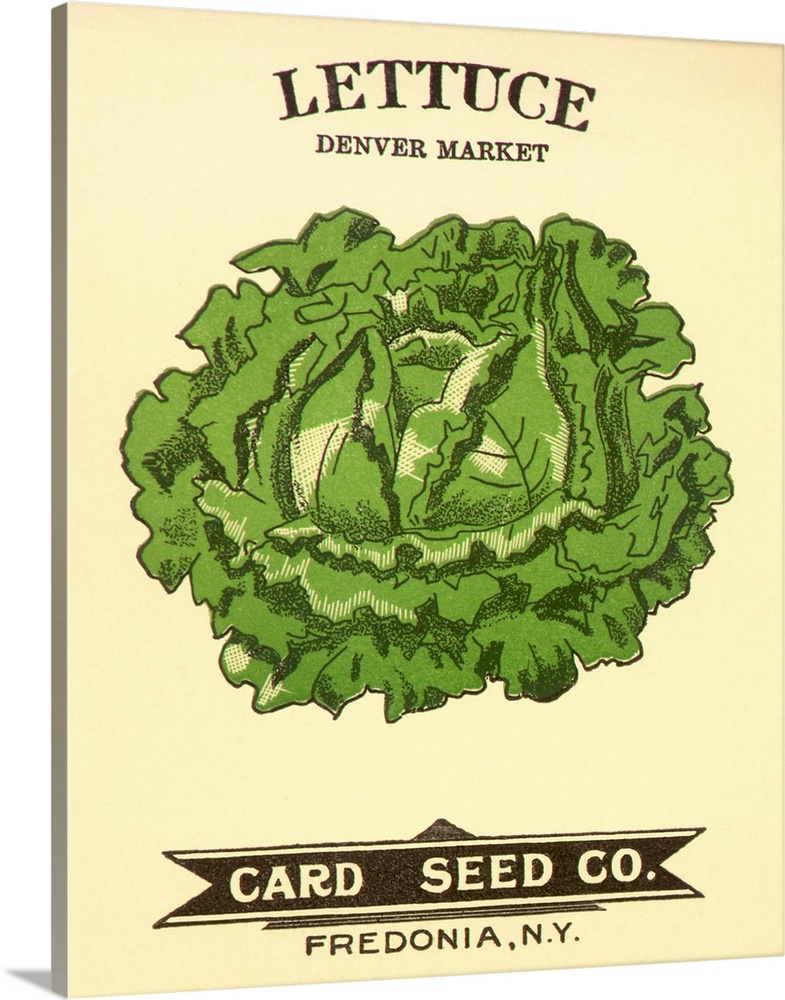This illustration depicts a vintage seed packet for "Lettuce, Denver Market" against a light grayish-yellow background. At the top, the label prominently displays "Lettuce" and "Denver Market" in brown and white lettering. Below this, a vibrant, cartoonish illustration of a lush, ruffled head of lettuce fills the center, showcasing a range of green hues with intricate darker shading and white highlights to convey texture and depth. Beneath the lettuce image is a brown ribbon banner that reads "Card Seed Co." in white text, matching the yellowish tone of the background. Below the ribbon, the text "Fredonia, N.Y." is printed in a straightforward manner. A brown triangle peeks out just above the word "Seed," adding a subtle design element. The overall aesthetic of the image evokes a sense of nostalgia, suggesting it is an old or vintage advertisement for the seed company, though the condition and quality indicate a possible modern reproduction.